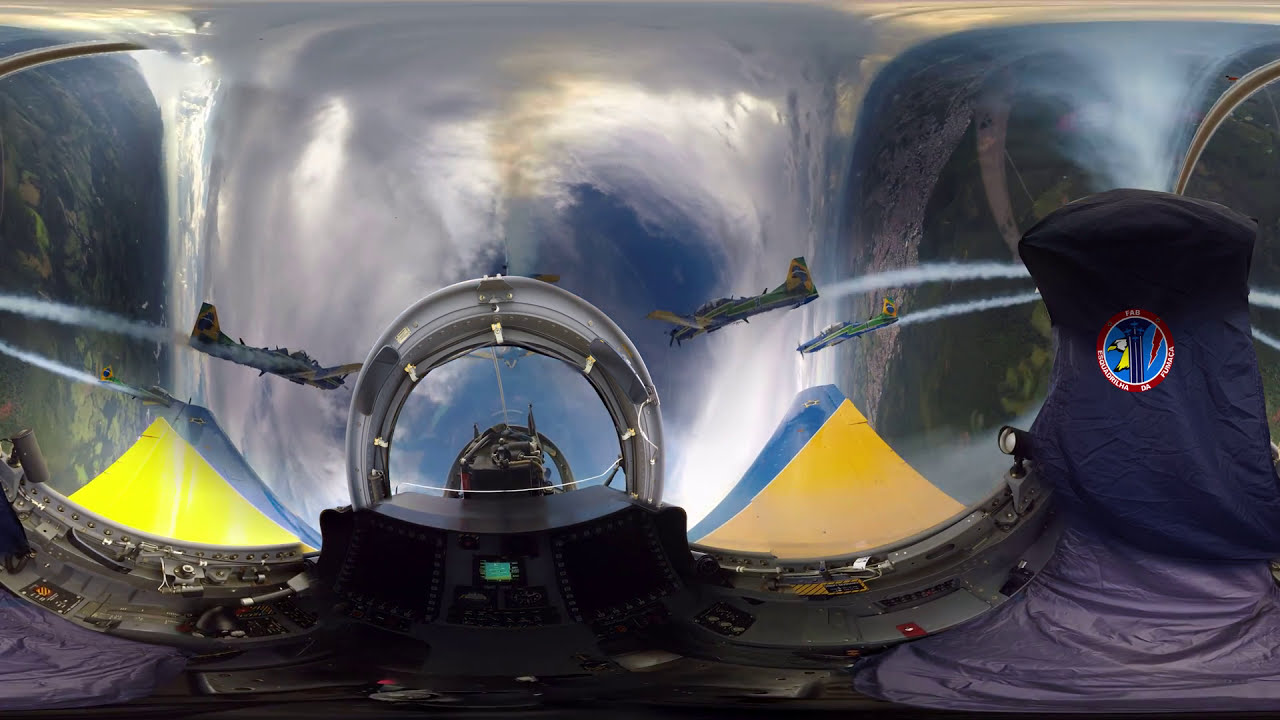The image captures a breathtaking view from within a vintage fighter plane, which appears to be upside down. The back of the pilot's head is visible, situated beneath a glass canopy that covers both occupants of the plane. The plane's wings, painted blue and yellow, are prominent. Outside, four other planes, seemingly older models with distinctive tail rudders, fly in formation, all heading in the same direction. On the right side of the image, an icon featuring an eagle, a plane, and a red lightning bolt is attached to the interior. The aircraft's instrumentation is partially visible, including a prominent black box with a green screen in its center. Outside the canopy, the ground below is green, dotted with clouds, creating a visually captivating scene of a military jet maneuver.